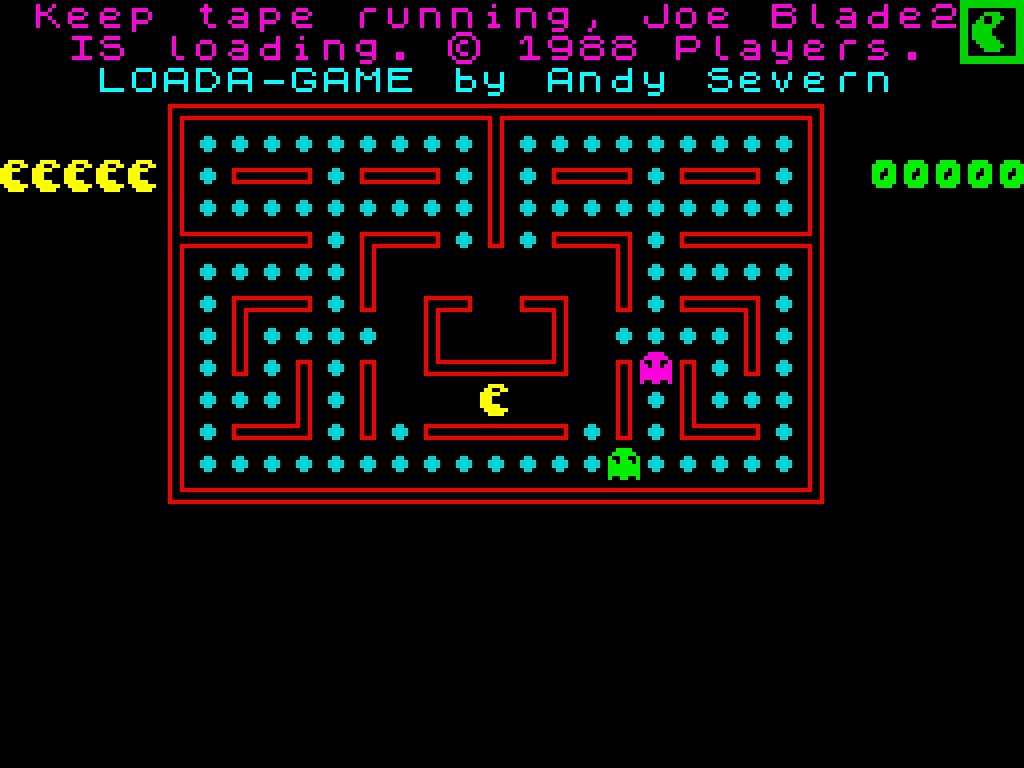This image is a screenshot of the classic Pac-Man arcade game. The game is displayed against a black background, featuring a maze outlined in red. Within the maze, small blue dots are scattered, which Pac-Man aims to eat. Notably, Pac-Man is being chased by two ghost characters—one is green and the other is a bright magenta color.

On the left-hand side of the screen, five Pac-Man symbols are arranged vertically towards the top, indicating the remaining lives. There are also five green power pellets in the maze, signifying special items that Pac-Man can consume for temporary advantages. 

At the top of the screen, there is text in a magenta color that reads, "Keep tape running. Joe Blade 2 is loading," followed by a copyright notice: "© 1988 Players." Further below, light blue text states, "Load-game by Andy Severin," providing credit to the game developer.